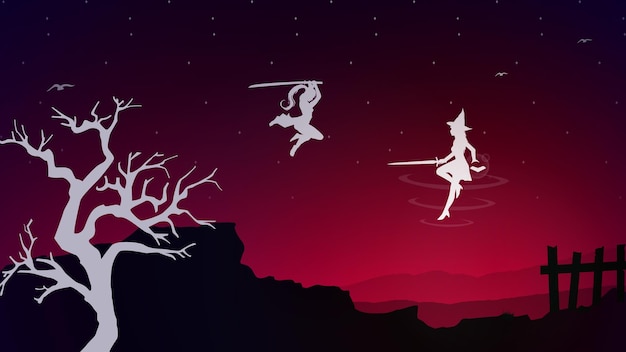In a striking, reddish sky that darkens to a black, starry dome above, an intense scene unfolds. A landscape of rocky ledges and eerie elements is bathed in this vibrant hue, with a stark white, gnarled tree standing prominent on the left. This barren tree stretches down to the bottom of the frame. To the right, a broken wooden fence with four posts adds to the desolate ambiance.

At the center of this vivid backdrop, suspended in mid-air, is a silvery-white silhouette of a witch. She wears a pointy cap and a short dress, extending down to mid-thigh. In her right hand, she brandishes a sword pointed forward, while her other hand clutches a book. Spirals of red energy encircle her.

Above and slightly to the left of the witch, another white silhouette floats in a dynamic pose. This figure, adorned with a long ponytail and a cape, holds a sword aloft, seemingly poised to strike. Her legs are tucked beneath her as if she has leaped into the air, heightening the drama. 

Below this dramatic confrontation lies a jagged, black mountain range. To the far right, near the bottom of the frame, is a small, four-post fence, painted in the same black hue as the mountains. The sky around them transitions from the vibrant red horizon to the upper reaches of the black, starry firmament, dotted with tiny white stars. White silhouettes of birds or bats add to the gothic atmosphere of this fantastical scene.